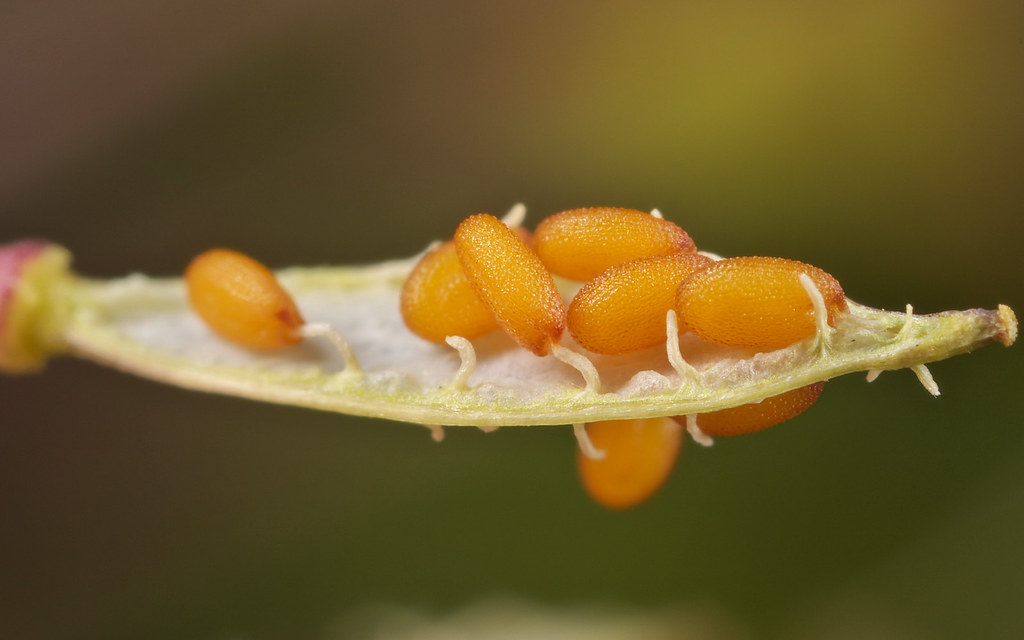This is a detailed close-up photograph of an unusual fruit. The fruit is connected to a plant and consists of several small, oval-shaped, orange seeds that look like miniature blimps or jelly beans. These seeds, having a rough yet almost translucent surface, are firmly attached to thin white filaments sprouting from the fruit. The fruit itself is green, resembling the shape of a tree leaf—broader in the middle and tapering towards the ends—with a darker yellow center. The background is a blend of blurry shades of green, fading into pink and red hues, adding a vibrant contrast to the focused details of the fruit and its seeds.